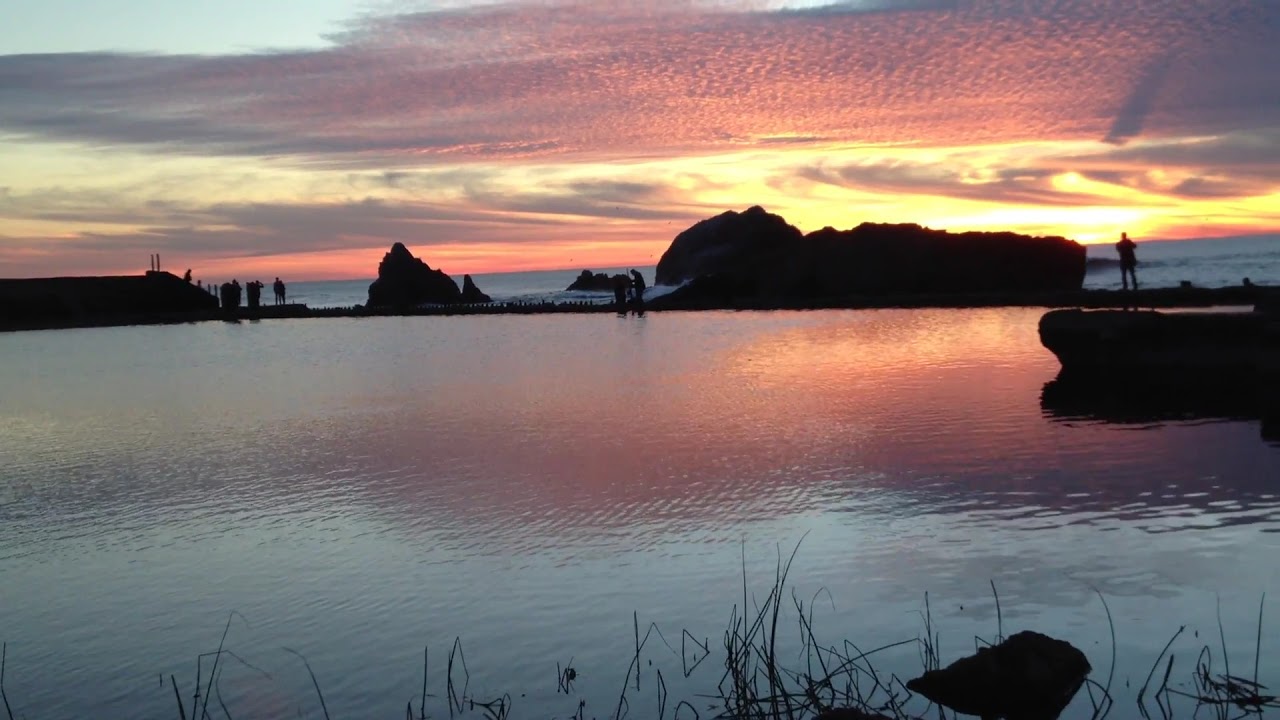This outdoor image captures a tranquil scene at either sunrise or sunset, featuring a serene lake or bay that reflects the stunning sky above. The bottom half of the photo showcases blue water, tinged with orange hues from the sky's reflection, and is punctuated by strands of grass emerging through the water. At the midpoint of the image, a row of dark boulders and possibly piers, populated with the silhouettes of people, serves as a barrier separating the still water from a thin strip of what appears to be ocean beyond. On the right, a rocky outcrop extends into the water, where another silhouetted figure stands. The sky occupies the top half of the picture, aglow with swirling clouds in vibrant shades of yellow, orange, and red, emanating from a hidden sun positioned in the lower right quadrant. The entire scene is bathed in the ethereal light of either dawn or dusk, adding a magical quality to the landscape.